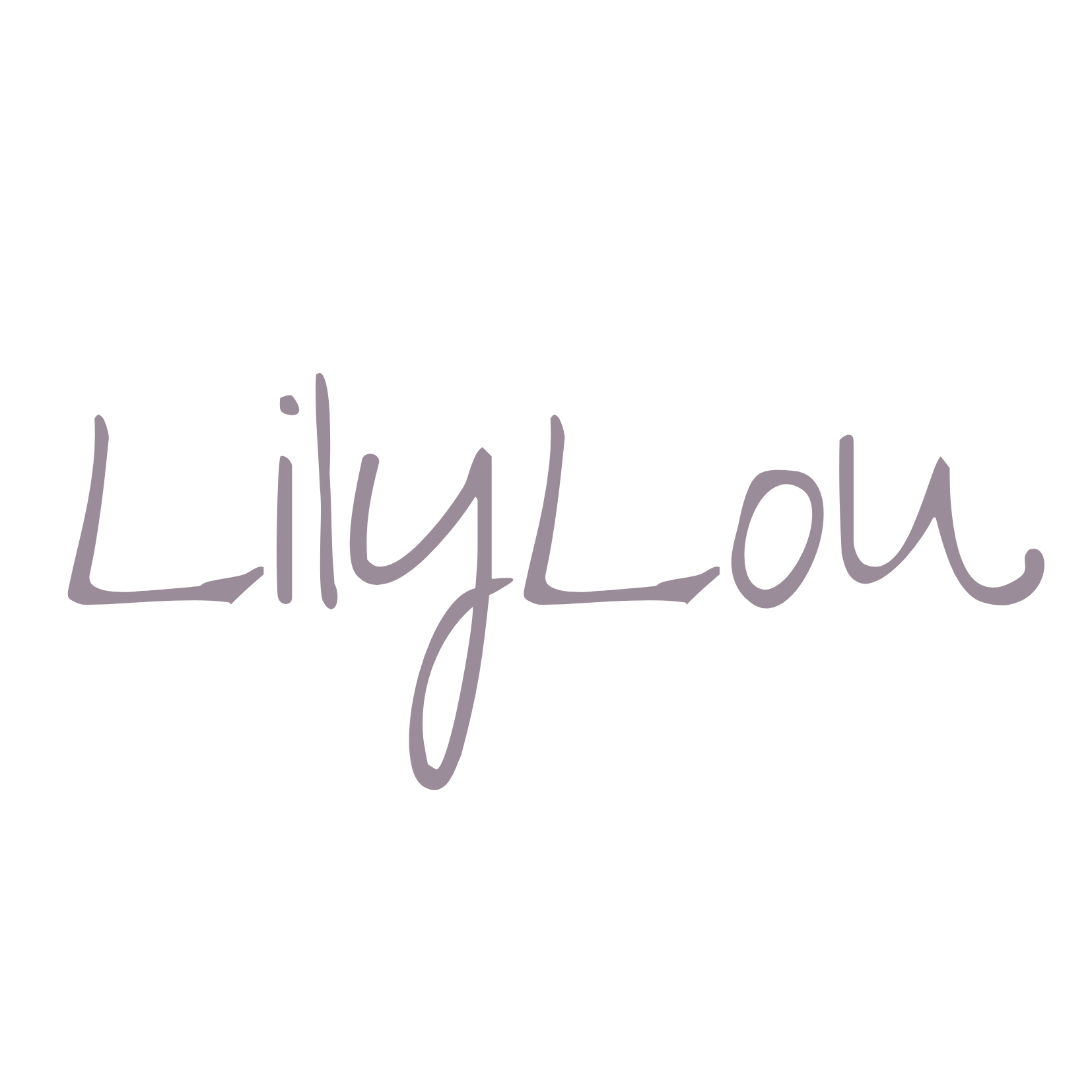In the image, a single name, "Lily Liu," is flawlessly handwritten in a stylish cursive script that is centered against a plain white background. The text is presented in a dark gray color, with notable details including both 'L's being capitalized and the tail of the 'Y' in "Lily" elegantly crossing itself to the right. The 'U' in "Liu" curves outward to the right, adding a distinctive touch. The font used is more sophisticated than standard text like Arial, yet not overly ornate. The simplicity of the image draws attention solely to the name "Lily Liu," which is positioned prominently in the center.